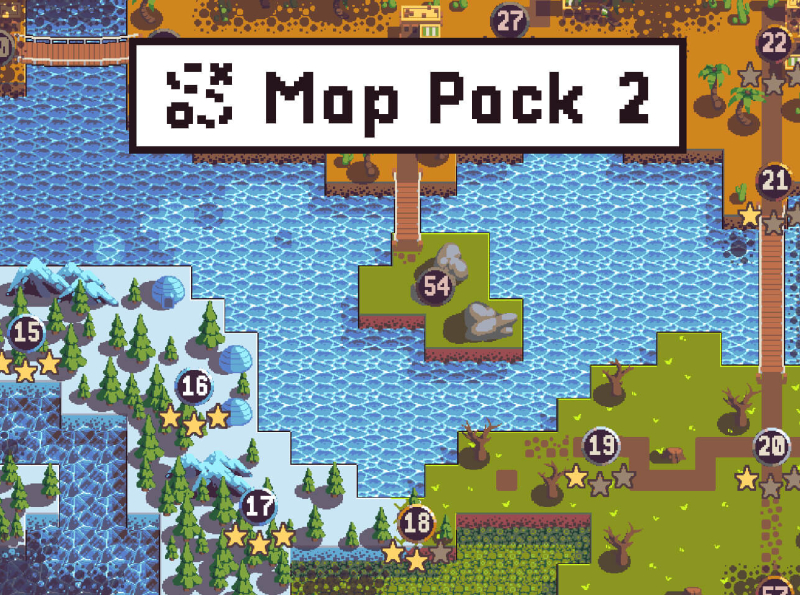This image is a detailed screenshot from a retro, pixelated video game with a 16 or 32-bit graphic style, viewed from a third-person, top-down perspective. At the center of the screen, prominently displayed in very pixelated text, is the title "Map Pack 2." Surrounding this central label, the map is divided into distinct landscape zones, each with unique characteristics and labeled with numbers in circular icons representing levels.

In the top portion of the image, there's a desert or beach landscape with sand and small palm trees. The ocean occupies the central area, and bridges, depicted as brown lines, span between landmasses. To the bottom left, there's a wintry region adorned with pine trees and igloos, set against a snowy white background, featuring the numbers 15, 16, and 17. The bottom right showcases a verdant field with leafless trees and a green base, where the numbers 19 and 20 are located.

Stars indicate the completion status of each level: golden stars are shown underneath the numbers, with up to three stars possible per level. For instance, level 16 features three golden stars, while level 19 exhibits one golden star and two grayed-out stars, hinting at incomplete achievements. The scattered numbers, such as 18, 20, 22, and 27, further report a comprehensive level structure across the different terrains, summarizing progress and challenges in this nostalgic gaming environment.